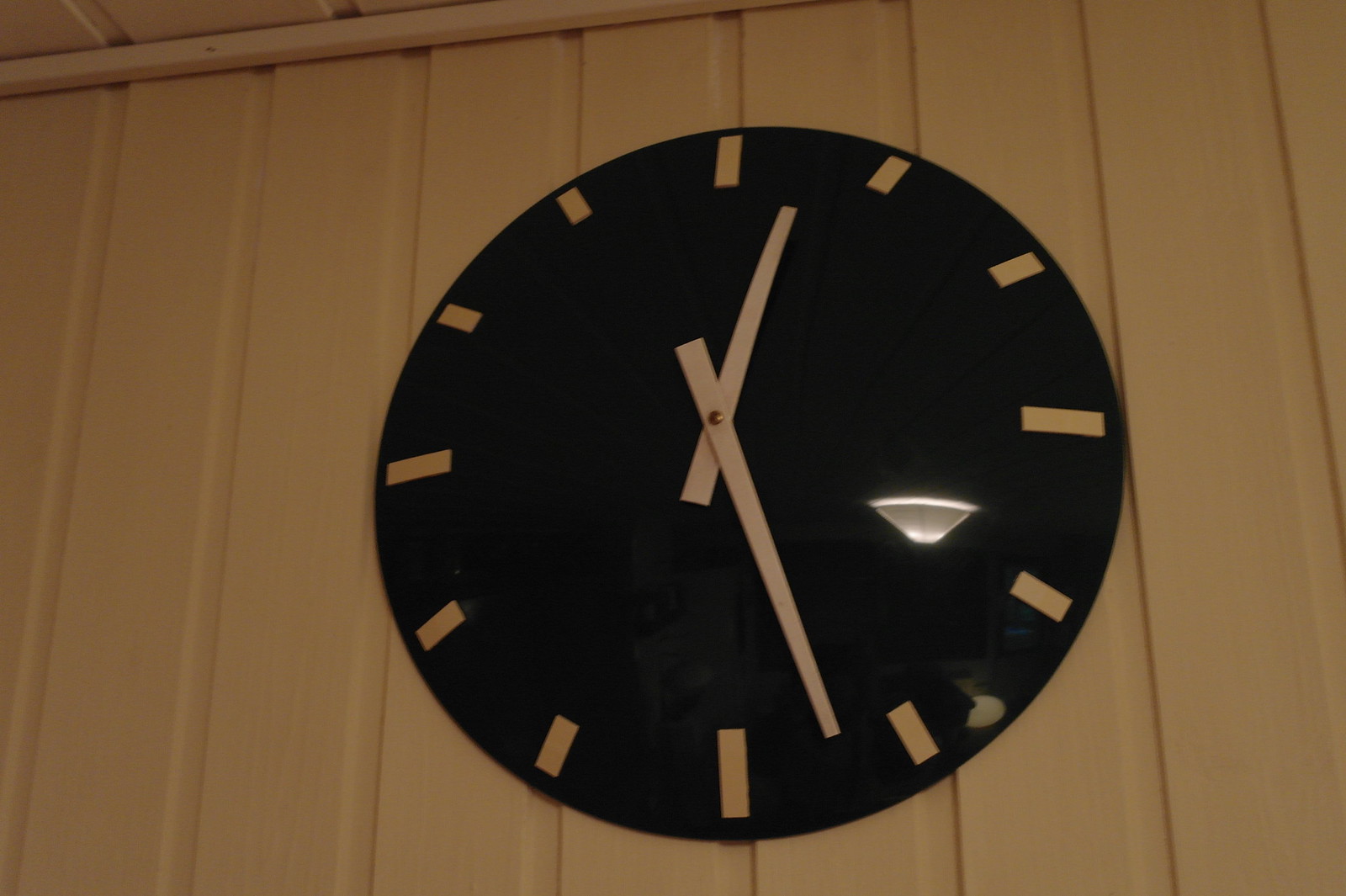In this photograph, we see a sleek, shiny black round analog clock mounted on a textured, corrugated metal wall that has a dull pinkish beige hue. The clock itself resembles a slightly rounded yet flat disc, akin to a Frisbee, with a glossy finish that hints at a plastic or glass material. Instead of numbers, the clock face features small rectangular dashes to indicate the hours, with slightly longer rectangles marking the 12, 3, 6, and 9 positions. The hour and minute hands are elongated, narrow pink rectangles matching the dash markers. A notable white light shines through the clock's transparent edge, and the clock is prominently set against the backdrop of panel-like wall siding, hinting at possibly being in an outdoor or industrial area.